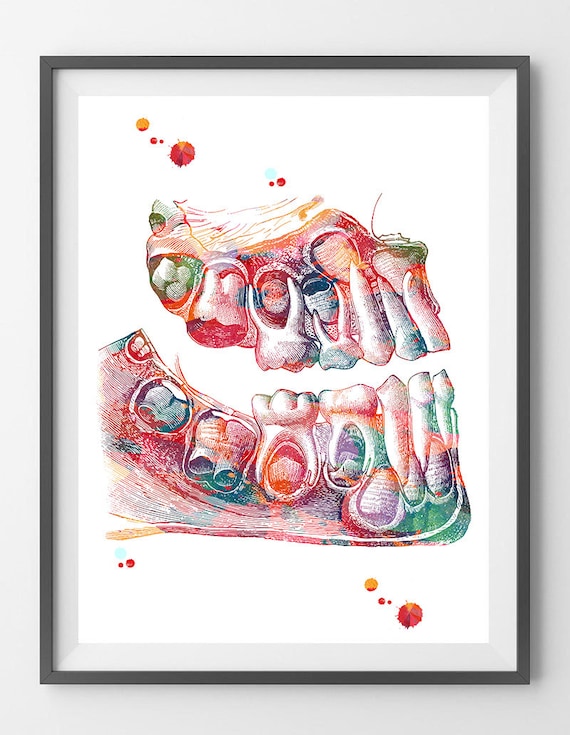The image shows a vibrant and stylized piece of artwork, framed in a black rectangular frame with a light gray matting about an inch wide surrounding it. The artwork itself, set against a stark white background, depicts a detailed side profile of a human jaw with exposed teeth. The image, drawn with what appears to be pen and ink, highlights the teeth and their roots, using an assortment of muted yet vivid colors such as greens, purples, reds, and oranges. The front teeth, located toward the center right of the image, are predominantly green, while the colors transition to reds and other hues as they move towards the back molars on the center left. Drops of ink can be seen above and below the jaw, adding to its artistic flair. The teeth are shown in various stages of development; some are clearly visible, while others, particularly the back molars, are still nestled within the gums. The image captures an anatomically revealing and aesthetically intriguing examination of a human jaw.